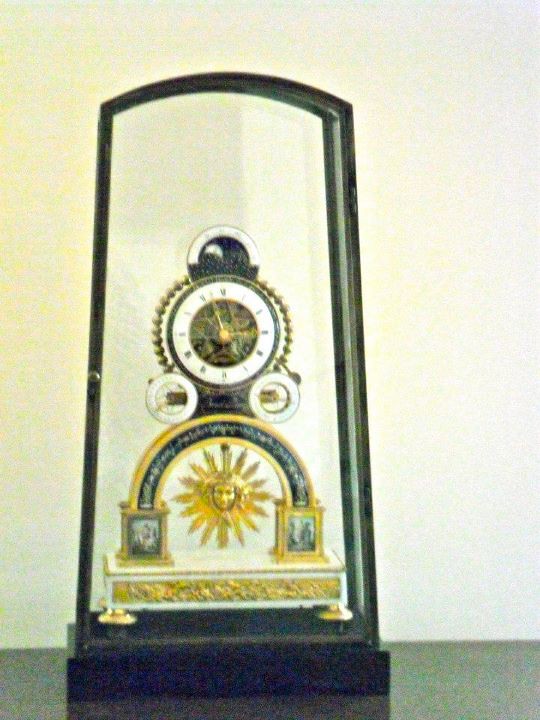The image features a tall, ornate clock with a black arched frame sitting on a charcoal gray, rectangular base. The base itself is detailed with gold inlay and stands on short gold legs. The clock face is round and white, surrounded by a loop of gold beads resembling a chain, and is hard to read due to the image's low resolution. The clock hands are gold, and the face displays black numbers, possibly reading 3:57 or 11:15. Above the clock face, there's a semicircle centerpiece with a sunburst design featuring a sun with a human face. This semicircle includes multicolored dark red, yellow, and black elements, likely representing a sky with white star-like dots. The entire structure exudes an antique, bronzy gold allure, set against an off-white wall, giving it a grandiose, intricate appearance.